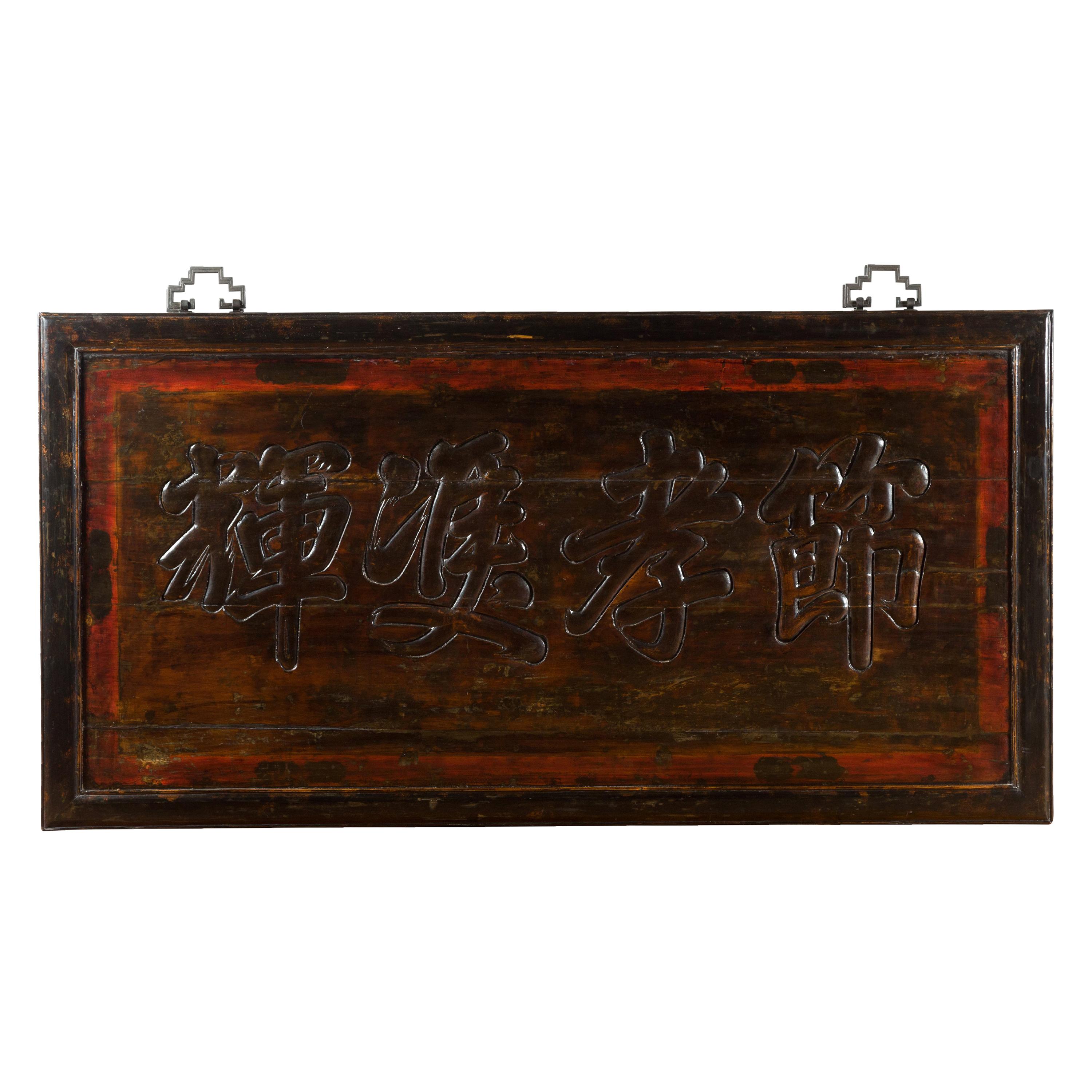The image depicts a very old, rectangular wooden plaque set against a stark white background. The plaque itself features a dark brown exterior with a faded, reddish-orange interior that highlights a central wooden square. This square is adorned with four large, hand-carved Asian characters, likely Japanese, Chinese, or Korean in origin. The characters display a distinct texture, differentiating them from the rest of the plaque's smooth, glazed surface. The top of the plaque has two silver hinges with intricate, staircase-like patterns, indicating it may have been part of a box or a hanging piece. The overall appearance is aged and slightly worn, suggesting a rich historical significance.